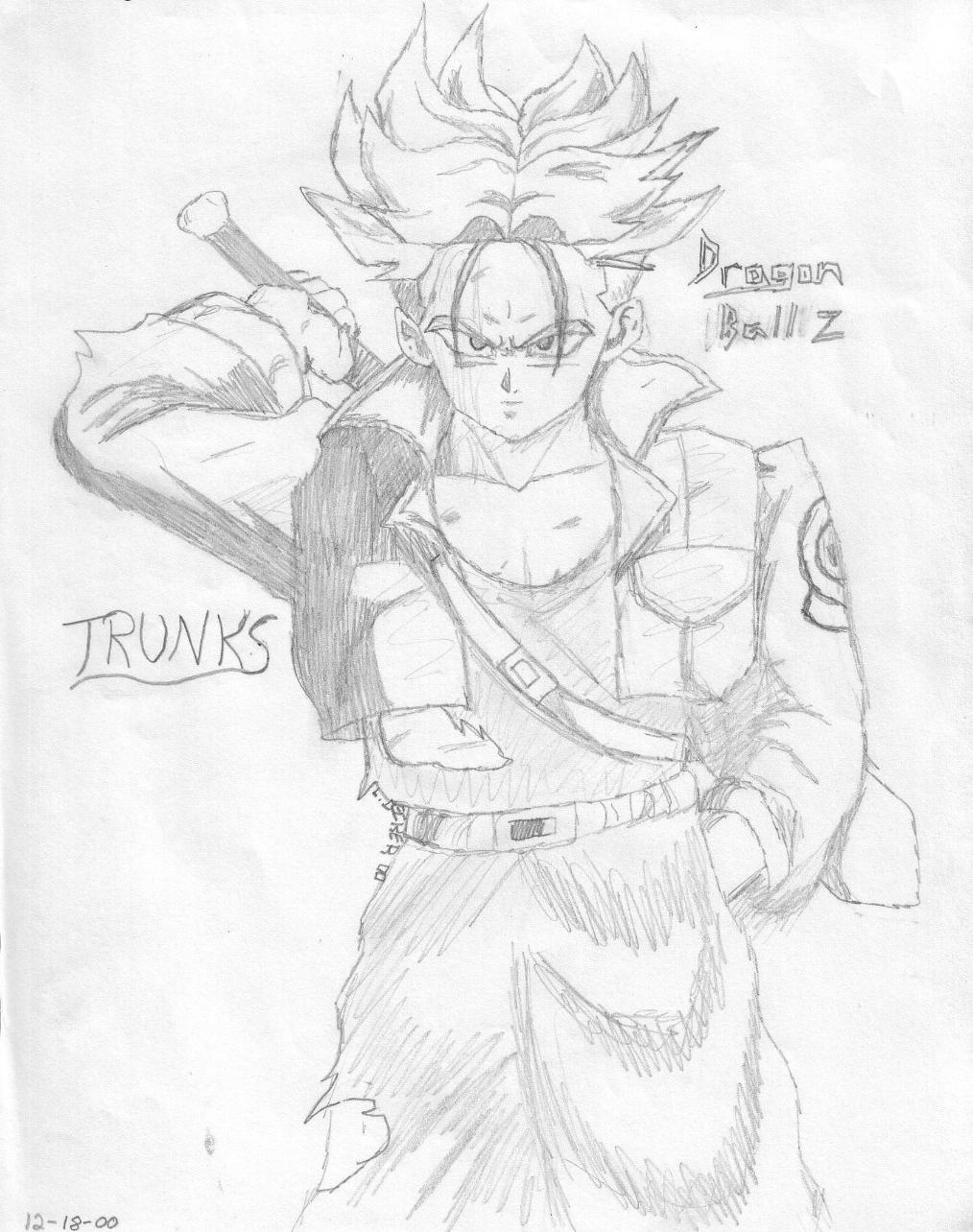This detailed sketch from December 18, 2000, is fan art of Future Trunks from Dragon Ball Z. Drawn on a piece of white paper with pencil, the character is depicted in an intense and dynamic stance, capturing the essence of his Super Saiyan transformation. Trunks' unmistakable spiky blonde hair is parted in the middle, flaring upward with two strands falling on his face. His eyes convey a determined and focused expression. 

He is clad in a heavily detailed outfit: a shortened jacket with the Capsule Corp logo, a cross-body strap, a belt, and slightly ripped jeans. One hand is seen reaching behind his back to grasp the hilt of his iconic sword, while his other hand is casually tucked into a pocket. The word "TRUNKS" is prominently written beside his arm, and the title "Dragon Ball Z" is inscribed above his shoulder. The drawing includes small details such as a few wrinkles in the upper right-hand corner of the paper and the date clearly written in the bottom left corner. This artwork vividly encapsulates Trunks' readiness for battle and his role as a time-traveling warrior from a dystopian future.